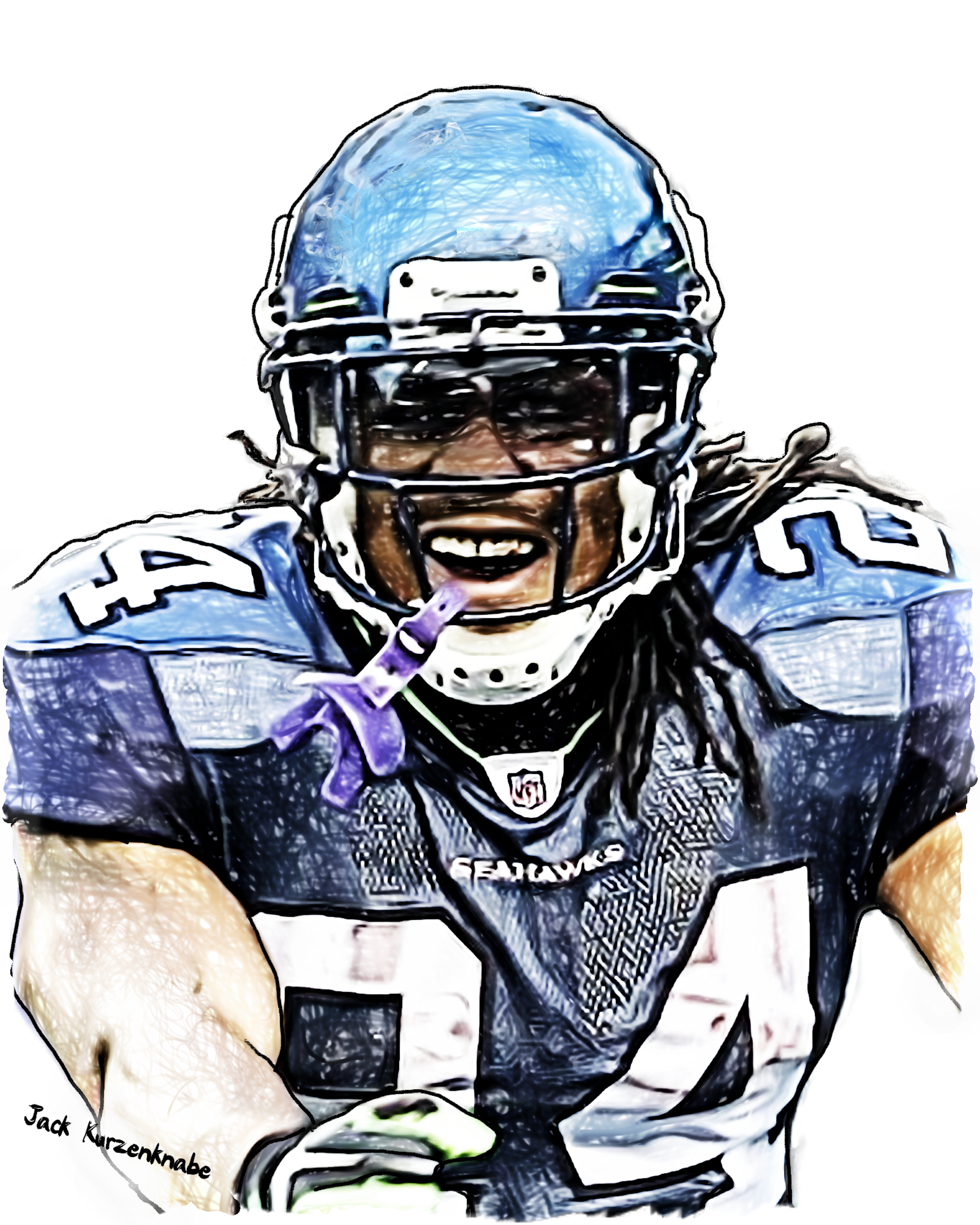This image is an artistically edited photo of an African-American football player, believed to be Seattle Seahawks' Marshawn Lynch. The photo is transformed using a sketch-like filter, which gives it a hand-drawn appearance with wavy, imperfect outlines. The player is seen in a dynamic pose, running towards the camera, with the background entirely white, emphasizing the focused zoom on the player's upper body.

The player is wearing a light blue and dark blue Seattle Seahawks jersey, featuring a white NFL logo with a black outline at the center. The jersey's number appears to be 24, inferred from the visible white '2' on the left shoulder and white '4' on the right shoulder, both outlined in black. Additionally, part of the number 24 is also discernible on the front of the jersey along with the word 'Seahawks' written in white.

He dons a light blue helmet and has a light purple mouth guard dangling from it. His right arm, featuring a glove, is in front of him on the left side of the image, while the other arm is cut off due to the tight crop of the image.

The bottom left of the image bears a stylized signature in black that reads "Jack Kurzenknabe," indicating the artist responsible for this depiction. The overall effect is a striking blend of photography and sketch artistry that captures the player's triumphant and dynamic spirit.